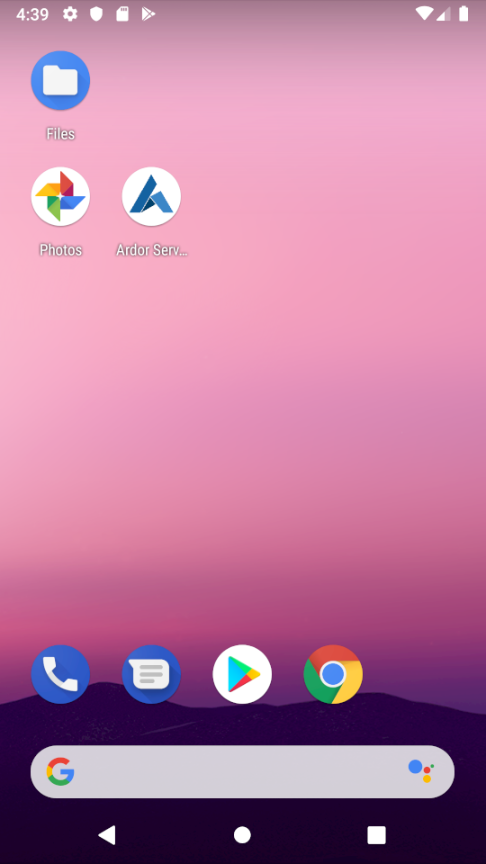The image features a phone screen with a visually striking ombre background. The background transitions from a bright, light pink at the top, gradually becoming a more vivid and darker pink as it moves downward. This pink hue then shifts into a purple, forming a gradient that fades into dark blue and, finally, black at the bottom, creating a serene yet dramatic effect. 

A mountainous or hilly landscape in dark purple silhouettes the bottom of the screen, blending seamlessly into dark blue and black. 

In the top left corner, there are various status icons in white: the time displayed as "4:39", a settings icon, a shield symbol, an SM card icon, and a play button pointing to the right. 

On the top right corner, there are connectivity indicators: the Wi-Fi signal, cellular bars, and a battery icon. 

Below this, three app icons are aligned in the top left corner. The first app is labeled "Files" and depicts a white file on a blue circular background. Underneath it, there is the "Google Photos" icon, labeled "Photos." Next to it is an app labeled "Adore Serve" with an arrowhead pointing upward, displayed in blue on a white background. 

At the very bottom of the screen, the navigation bar is visible: a play button pointing left on the left side, a circle icon in the middle, and a white square on the right side. 

Above the navigation bar is the Google search bar. Further up, there are four app icons aligned horizontally from left to right: the Phone icon, Messaging app, Play Store, and Google Chrome.